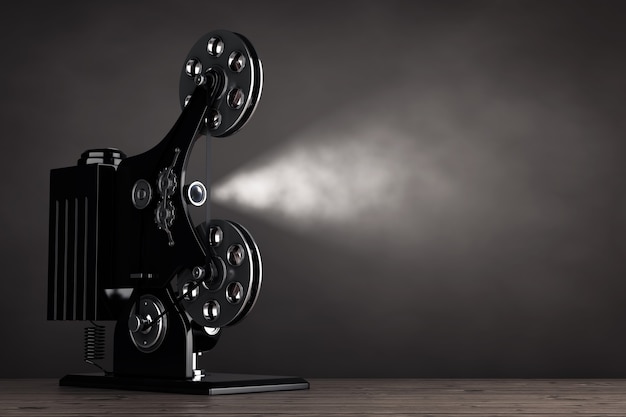This is a realistic, color photograph, oriented as a horizontal rectangle, depicting an old-time movie projector in a dark setting. The background is predominantly black, darker at the edges and slightly lighter in the center, drawing attention to the main subject. The bottom of the image features a dark wood surface on which the projector is placed. The sleek, metallic projector seems both antique and meticulously cleaned, suggesting it might have been digitally rendered or enhanced. It stands on a tall metal frame with silver stainless steel reels, designed to spool the film through the device. A conical beam of white light projects from the lens on the left side, cutting a triangular path across the image toward the right, creating a glowing gray cloud effect against the dim surroundings. The image is devoid of text, people, animals, buildings, or vehicles, focusing solely on the detailed and evocative representation of the movie projector.